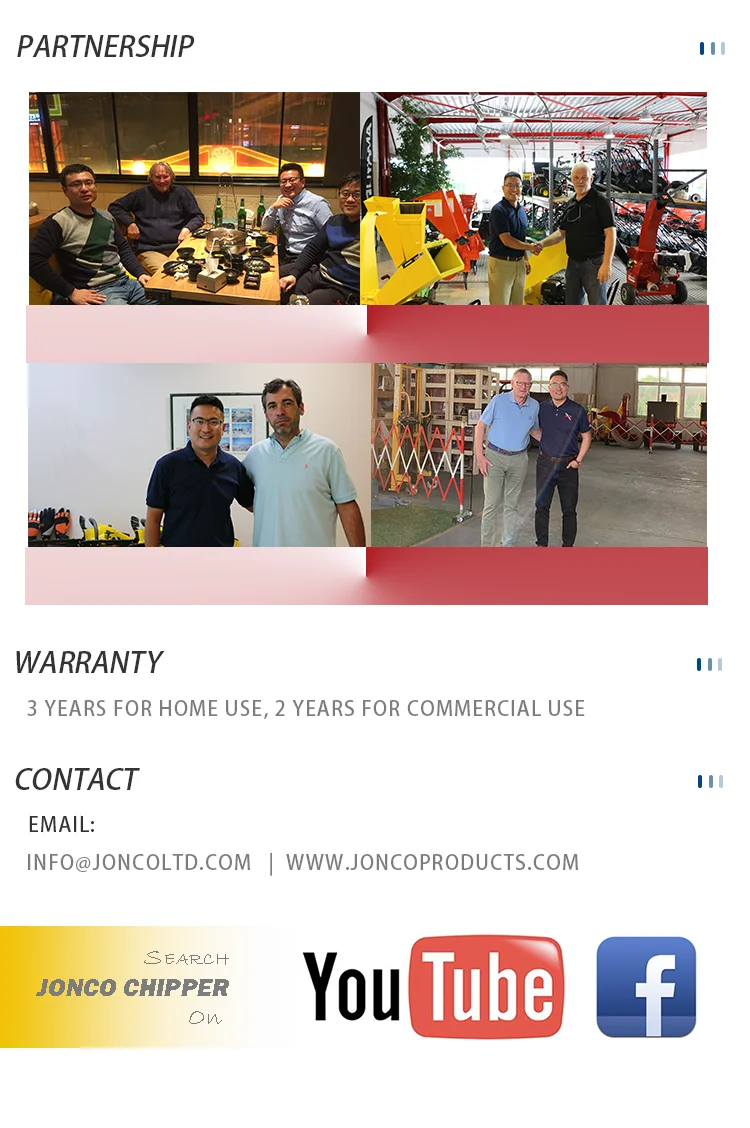At the top of this vertically rectangular web page, in the upper left corner, the word "PARTNERSHIP" is displayed in gray capital letters. Beneath this, a box containing four distinct photographs showcases scenes of camaraderie and teamwork, including two men either shaking hands, hugging with arms around each other, or sitting around a table in a communal setting.

Below this image box, the word "WARRANTY" is presented in gray capital letters. Directly underneath, in light gray capital letters, it states: "3 YEARS FOR HOME USE" and "2 YEARS FOR COMMERCIAL USE". Further down, the word "CONTACT" appears in light gray capital letters, followed by "EMAIL" also in capital letters. In very light gray capital letters, the email address "INFO@JOHNCOLTD.COM" and the website "WWW.JOHNCOPRODUCTS.COM" are listed.

At the bottom of the page, an orange rectangular box that transitions from bright gold on the left to white on the right contains black text reading "JOHN CO. CHIPPER OWNER". Alongside this text, YouTube and Facebook icons are positioned, indicating social media links.